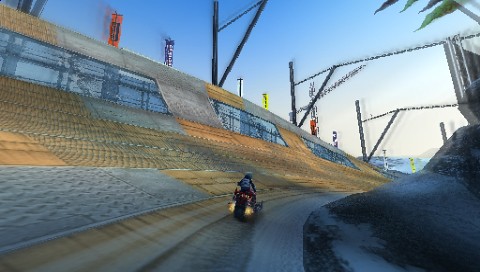A computer-generated image depicts a man riding a motorbike along a rugged track. The top part of the image showcases a clear blue sky, with the upper right corner adorned by the edges of some vibrant green leaves. Descending from the top left corner is a prominent structure, characterized by horizontal yet downward-sloping lines, extending almost to the image's center. This structure, featuring a blend of brown and gray hues, has rectangles cut out near its top and slightly slopes inward at the bottom. Below this formation runs a narrow track, similarly colored in shades of gray and brown. At the center of the track, the back of the motorbike rider is visible, positioning towards the right. The bottom right corner of the image reveals a rocky protrusion, textured in a blend of gray and black tones.